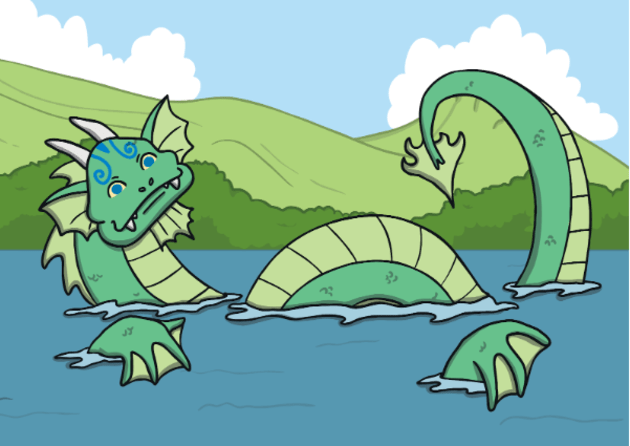The image is a vibrant, cartoonish illustration likely intended for a children's book. It features a seafoam green dragon with light green accents relaxing in teal blue water, with its head, belly, curved tail, and one of its front and back feet protruding from the surface. The dragon, which also resembles a Loch Ness Monster, floats on its back, gazing up at the sky. Its distinctive features include white horns, blue eyes, white fangs, and a small triangular-shaped sphere at the tip of its tail. It also has blue accent curls on its forehead. The background showcases green hills and lush greenery, with a clear blue sky dotted with a few fluffy white clouds on either side. The overall style is whimsical and enchanting, enhancing the fantastical atmosphere of the scene.